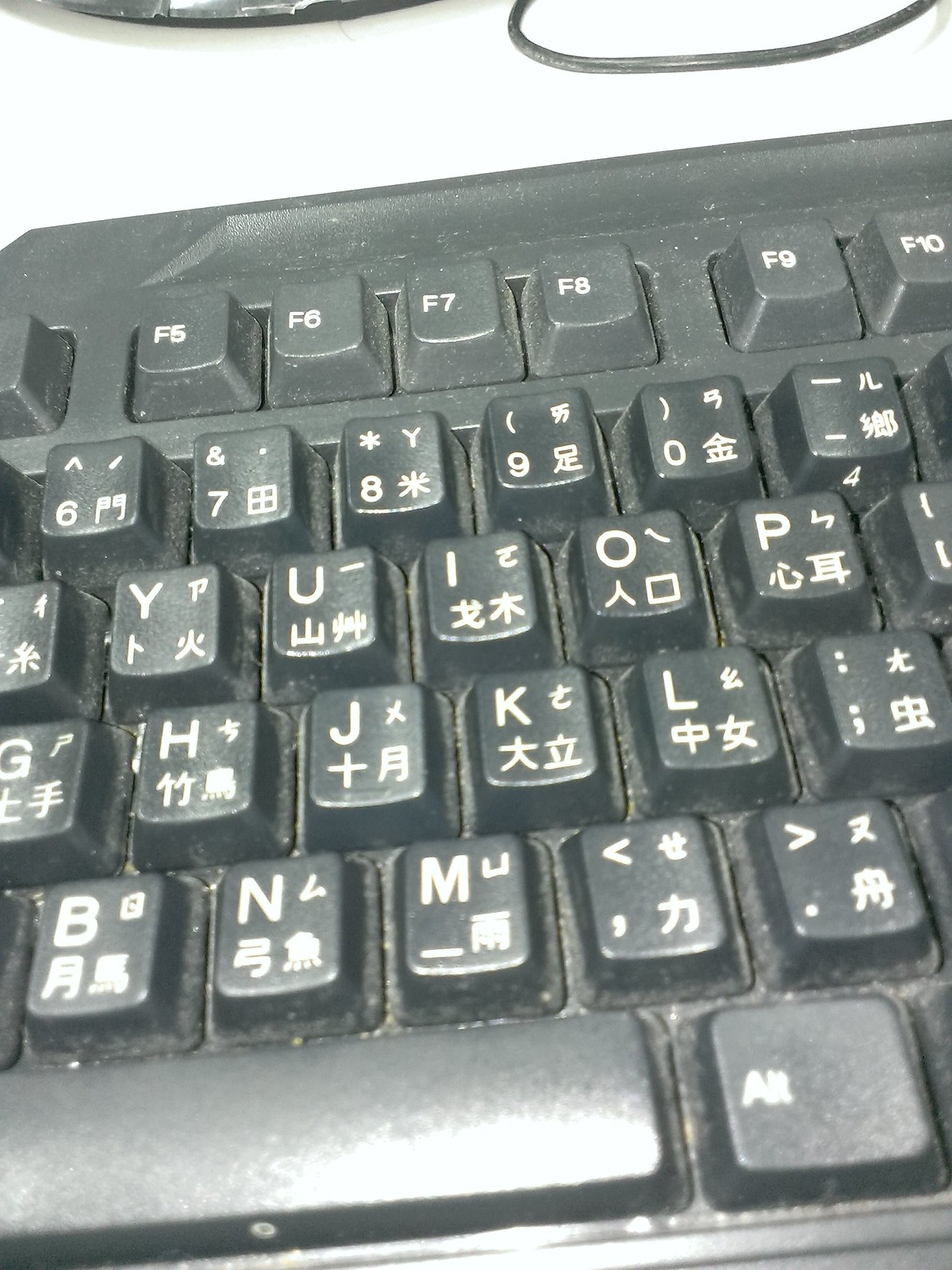The image depicts a zoomed-in, close-up view of a black mechanical keyboard placed on a white table. The keys are a combination of Latin characters and Japanese, suggesting it is for a Japanese speaker. The sections visible include the standard function keys (F5-F10), numbers 6 through 0, some letter keys such as Y, U, I, O, P, and G, H, J, K, as well as part of the spacebar and the Alt key to the right of it. Notably, the keyboard appears quite old and is in poor condition, with a considerable amount of dust and dirt accumulated both on and between the keys, and the letters appear faded. There is a cord visible at the top part of the image, possibly from a connected device like a mouse. The keys are illuminated by a reflected light, likely from a flashlight, enhancing the visibility of the debris and the wear on the keyboard.